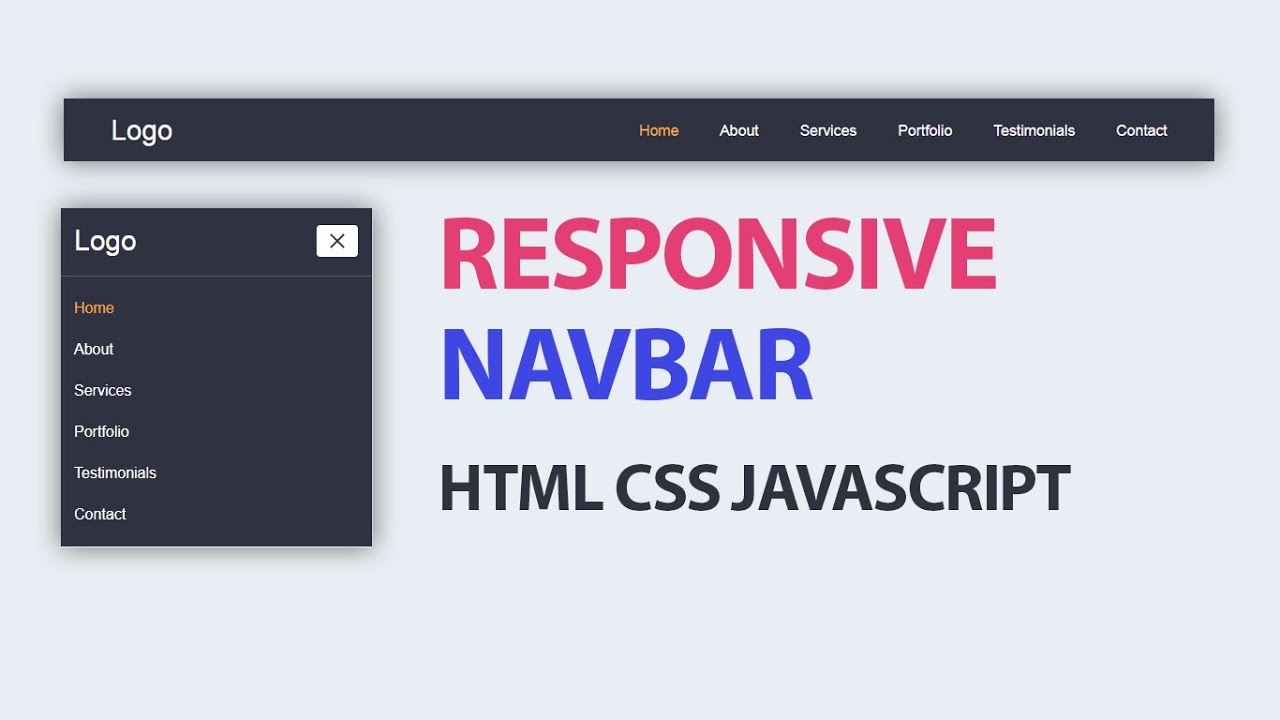The image depicts a sleek, modern website homepage layout. At the top, there's a navigation bar with a "Logo" placeholder on the top left. The navigation bar features the following tabs, each labeled in white text except the "Home" tab, which is in orange: Home, About, Services, Portfolio, Testimonials, and Contact.

Below the navigation bar, the background is predominantly white. On the left side of the image, there's a black sidebar with another "Logo" placeholder at the top, followed by an orange "Home" tab and white tabs for About, Services, Portfolio, Testimonials, and Contact. In the top-right corner of the sidebar, there's an "X" icon, suggesting a close or collapse function.

To the right of the sidebar, the main content features text descriptors in different colors. At the top, the word "Responsive" is displayed in red. Directly below it, "Nav Bar" appears in blue. Further down, the words "HTML, CSS, JavaScript" are listed in black.

Overall, the image highlights a clean, organized design utilizing a responsive sidebar that complements the top navigation bar, focusing on essential navigation elements and coding languages.